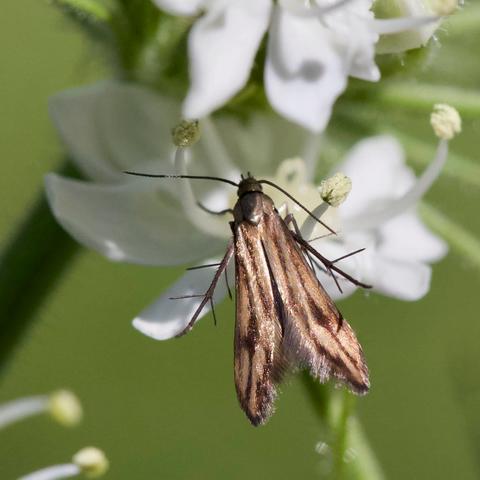This close-up photograph, set against a blurred green background, features two prominent white flowers with thin, widely spread petals. Each flower displays string-like stamens tipped with yellowish-cream pollen. Below the flowers, a robust, light green stem is visible. The focal point of the image is a brown moth perched on one of the flowers. The moth has folded wings with a darker brown pattern, a black head, long black antennae, and black-brown legs. The scene captures the moth amidst the delicate stamens of the flower, beautifully highlighting the interaction between the insect and the plant.